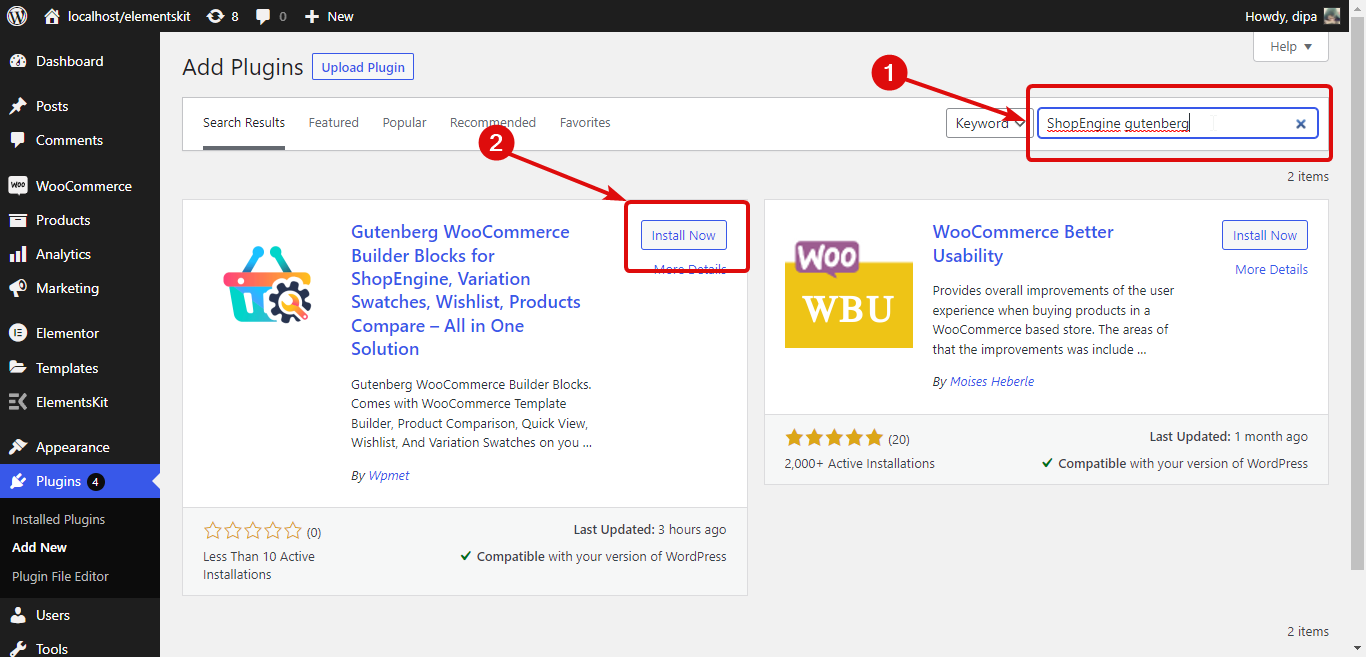The image displays a web dashboard interface with a black border at the top. On the upper left corner, a home icon is accompanied by the text "localhost/elementskit". A vertical menu is situated on the left side, listing various sections: Dashboard, Posts, Comments, WooCommerce, Products, Analytics, Marketing, Elementor, Templates, ElementsKit, Appearance, Plugins, Users, and Tools. The "Plugins" section is highlighted in blue, indicating it is currently selected. Under "Plugins", the options "Installed Plugins", "Add New", and "Plugin File Editor" are listed.

To the right of the vertical menu, the main content area has a gray header. At the top of this area, there are options to "Add Plugin" and "Upload Plugin". Below these options, there is a search box where the text "Shop Engine" has been typed in. This search box is outlined in red with an arrow pointing to it, labeled "1".